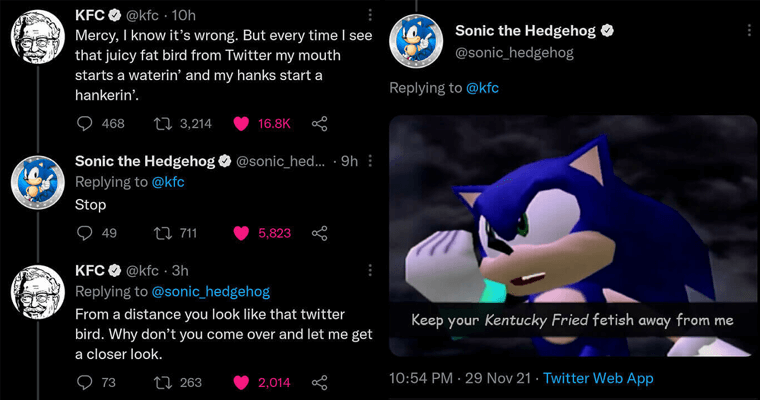**Screenshot of Twitter Exchange Between KFC and Sonic the Hedgehog**

The image is a screenshot of a Twitter conversation set against a black background. On the left, there is a black-and-white drawing of Colonel Sanders' face, accompanied by the verified KFC account (@KFC). The tweet reads: 

"Mercy, I know it's wrong, but every time I see that juicy, fat bird from Twitter, my mouth starts a-watering and my hanks start a-hankering."

This tweet has been retweeted 3,214 times, received 468 comments, and liked 16.8 thousand times.

In response, Sonic the Hedgehog (@Sonic_Hedgehog) replied with his blue avatar visible alongside the tweet:

"Stop."

This response has garnered 45 comments, 711 retweets, and 5,823 likes.

KFC then replies to Sonic with:

"From a distance, you look like that Twitter bird. Why don't you come over and let me get a closer look?"

This tweet has drawn 73 comments, 263 retweets, and 2,014 likes.

Finally, Sonic the Hedgehog, further responding to KFC with the same blue avatar, posts a picture of himself looking angry with his fist raised toward Colonel Sanders:

"Keep your Kentucky Fried Fetish away from me."

This last tweet was posted at 10:54 p.m. on November 29, 2021, via Twitter Web App.